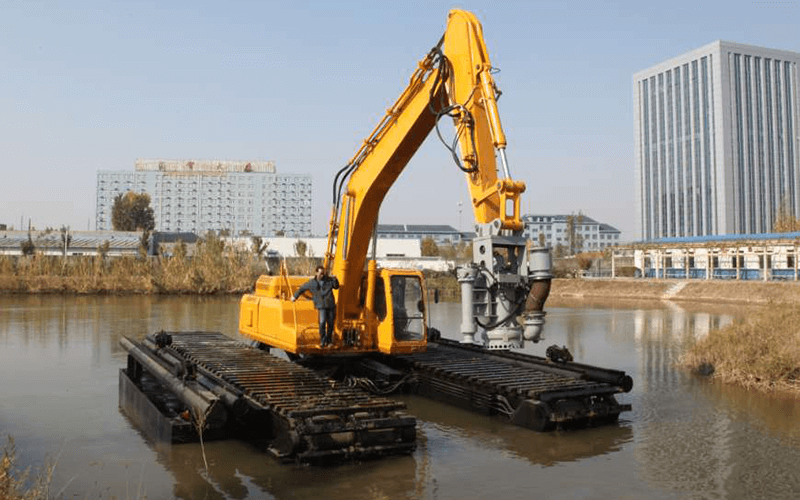The image shows a piece of heavy machinery, painted in a bright yellow, situated in a murky, muddy man-made body of water, potentially a small man-made lake. The machine is equipped with a crane arm that ends in a pressure-like gray contraption, possibly a pump, and it sits on two black tank-like tracks that have taken on a shiny appearance due to the water. A man is seen standing on the machine, specifically to the left of the control cab, either posing for or taking a picture. Surrounding the water, there are light tan marsh plants. In the background, a white-walled warehouse with a blue base is visible, along with a cube-like office building with multiple windows and a light blue apartment building.